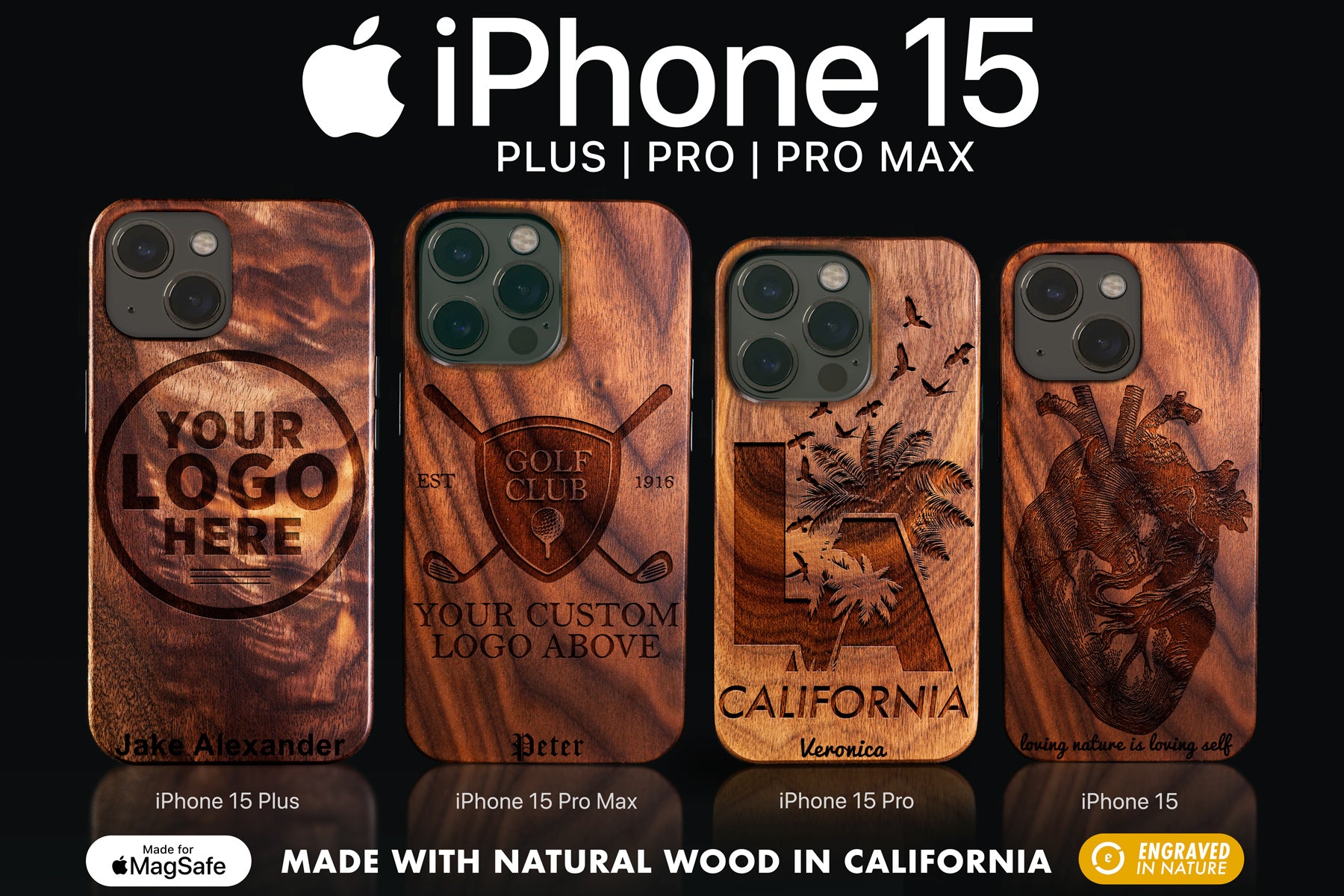The advertisement features iPhone 15 cases with a black background and a central white Apple logo accompanied by the text "iPhone 15" and the options "Plus, Pro, Pro Max" in white. Below this, four iPhones are showcased, each sporting a distinct wooden case engraved with unique designs. From left to right: 

1. **iPhone 15 Plus**: This case has a circle engraving reading "Your Logo Here" with the name "Jake Alexander" at the bottom.
2. **iPhone 15 Pro Max**: This features a coat of arms design labeled "Golf Club, Established 1916," with space for a custom logo and the name "Peter" at the bottom.
3. **iPhone 15 Pro**: The case is engraved with a palm tree, birds, and "LA California," along with the name "Veronica" at the bottom.
4. **iPhone 15**: This case displays an anatomical heart with the phrase "Loving Nature is Loving Self."

At the bottom, white text reads "Made with Natural Wood in California," emphasizing eco-friendly craftsmanship and the premium quality of the materials used.